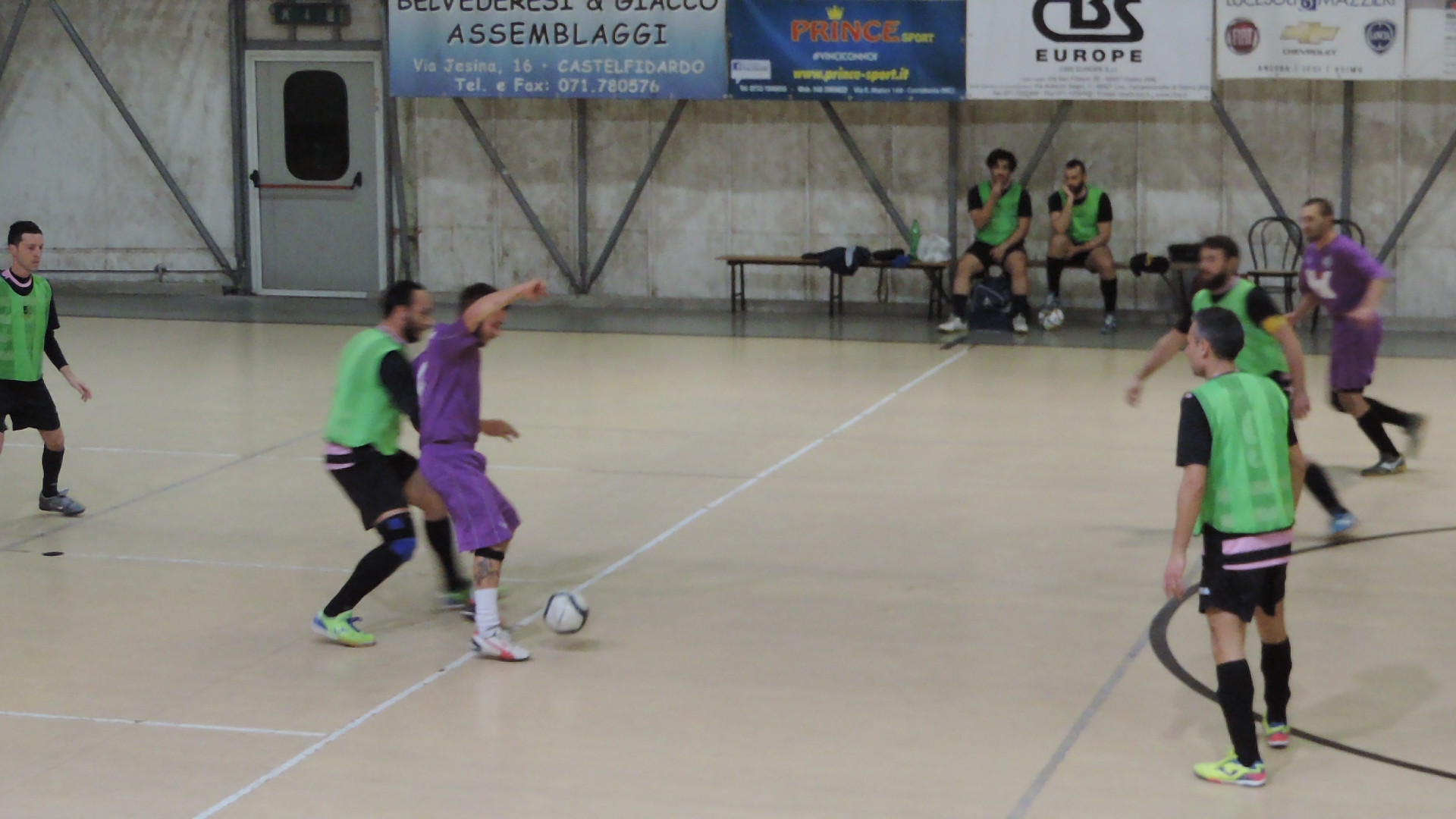The photograph depicts an indoor soccer game in a gymnasium with a tan-colored floor, likely a basketball court, and a white center line. The game pit players in purple uniforms against those in green vests over black shirts and shorts. On the left side, three players are visible: one in a green jersey closest to the edge, another green-shirted player near the centerline defending against a purple-uniformed player who has the ball by his right foot. On the right side, another three players are seen: two in green jerseys near the front and one in purple at the back. The wall in the background is gray cement, speckled and dingy, with a series of advertisement banners at the top—one light blue with black and white lettering spelling “ASSEMBLAGGI,” another darker blue with red lettering saying "Prince," followed by a white one with black text mentioning "Europe," and a fourth banner featuring company symbols including Chevrolet. There is also a gray metal door with a push bar on the left side of the image, and a low bench on the right with two seated players in green jerseys. The goalmouth and benches are visible, indicating a casual but active game setting.